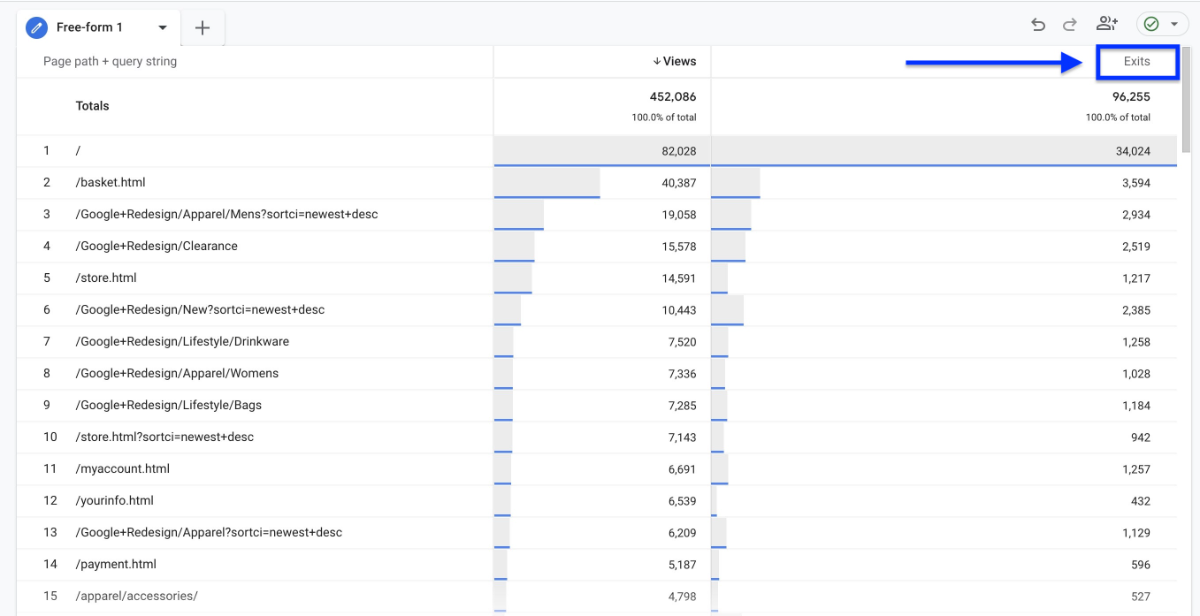Screenshot of a web dashboard showcasing traffic metrics for different HTML pages under the tab labeled 'Freeform'. The top left corner of the image prominently displays the 'Freeform' tab, indicating it is an editing interface for HTML websites. In the top right corner, there is an 'Exit' option within a blue rectangle, accompanied by a blue arrow pointing towards it.

The main focus of the screenshot is on two columns: 'Totals' and 'Views'. The 'Totals' column lists various pages starting with a simple backslash, followed by 'Basket HTML', 'Google Plus Redesign', 'Google Plus Redesign Clearance', and 'Store HTML'. The 'Views' column presents the number of views each page has received, with a combined total of 452,086 views. Specifically, the backslash entry has the highest individual count at 82,000 views, while 'Basket HTML' has 40,000, and 'Google Plus Redesign' has 19,000 views. The page with the least traffic is 'Apparel Accessories', registering just 4,798 views.

This screenshot appears to be an analytics dashboard summarizing website traffic, potentially indicating user engagement metrics for different web pages. The predominant source of traffic is noted to be the page listed as the backslash, although its exact nature isn't specified in the details provided.